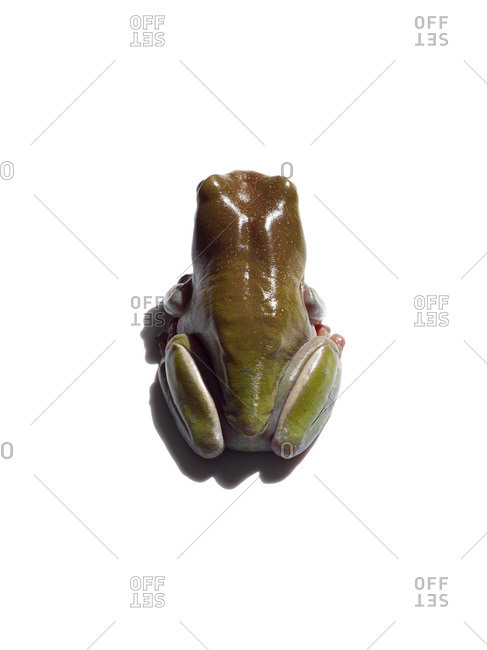The image depicts a frog viewed from the top, showing its richly colored back that transitions from a dark brown at the top of its head to a lighter brown on its back, and then to a greenish hue towards the lower part and on the tops of its legs. The frog's face is not visible as it is turned away, but its eyes seem to form noticeable bumps near the top of its head. Strikingly, the frog's back and head have shiny spots, indicating a light source from above.

The backdrop is a white solid background overlaid with large dashed gray lines, which create a diamond-shaped pattern. These lines intersect with the word "offset" arranged creatively within the diamonds; "OFF" appears normally while "SET" is inverted, with the letters for "S" and "T" mirrored vertically. The word "offset" and additional "zero" are repeated in certain segments of the background. The frog's limbs are tucked in, with the legs positioned upwards and the arms not clearly visible. Overall, the image presents a colorful and detailed view of the frog amid a structured yet artistic patterned background.